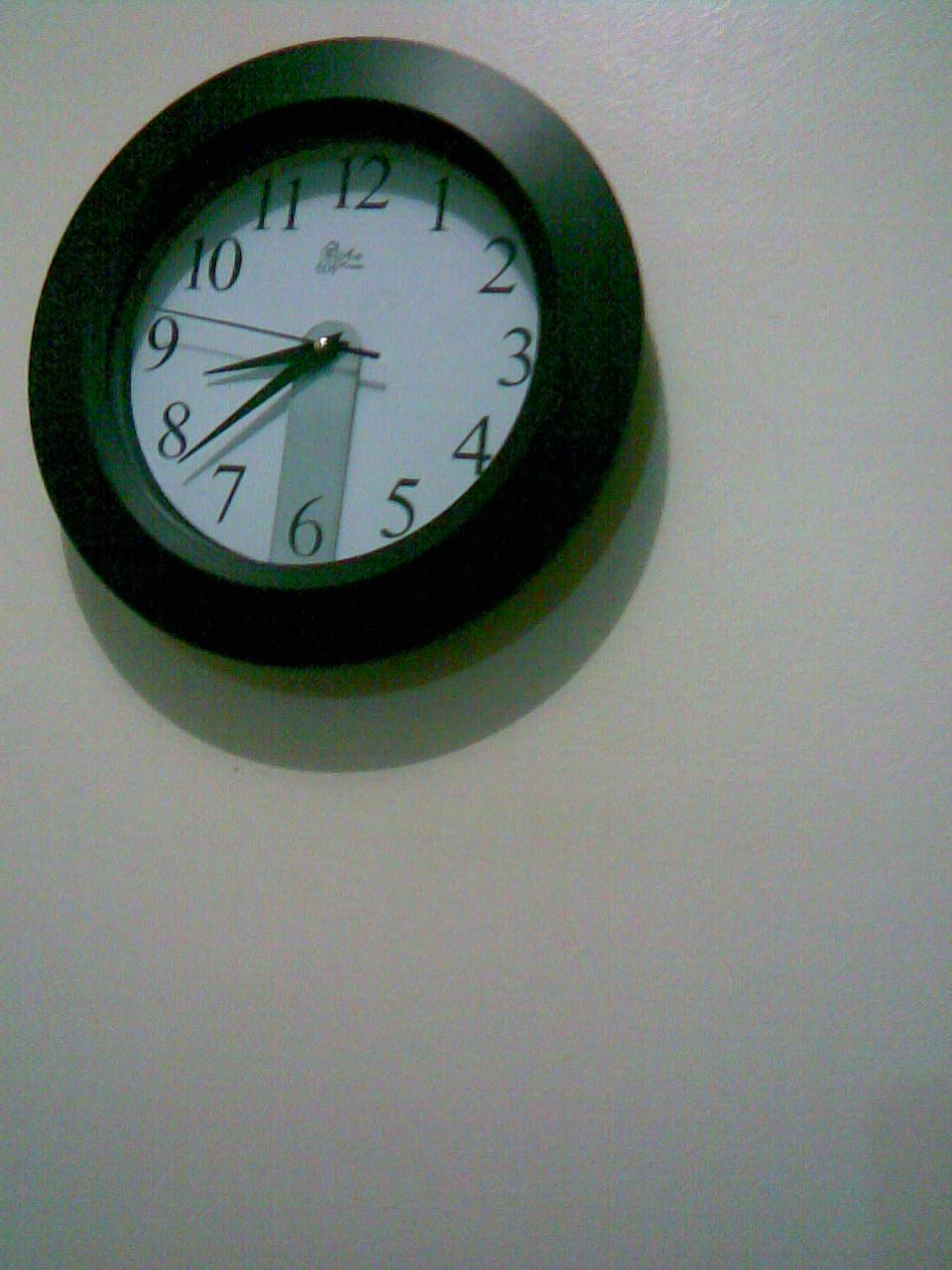This photograph captures a sleek, modern clock mounted on a pristine white wall, likely within an office building. The clock features a robust black frame encircling a classic white face. Traditional black numerals, starting from 12 at the top and continuing through to 11, mark the hours. Situated just below the number 12 is the clock's brand name, which is slightly ambiguous and difficult to discern. The clock's hands, including the second hand, are also black, and the time displayed is 8:37. A notable design feature is a darker gray segment extending from the number 6 to the central widget that secures the hands, adding a distinctive dimension to the clock's appearance. The clock casts a subtle shadow on the wall behind it, suggesting a light source from the side.